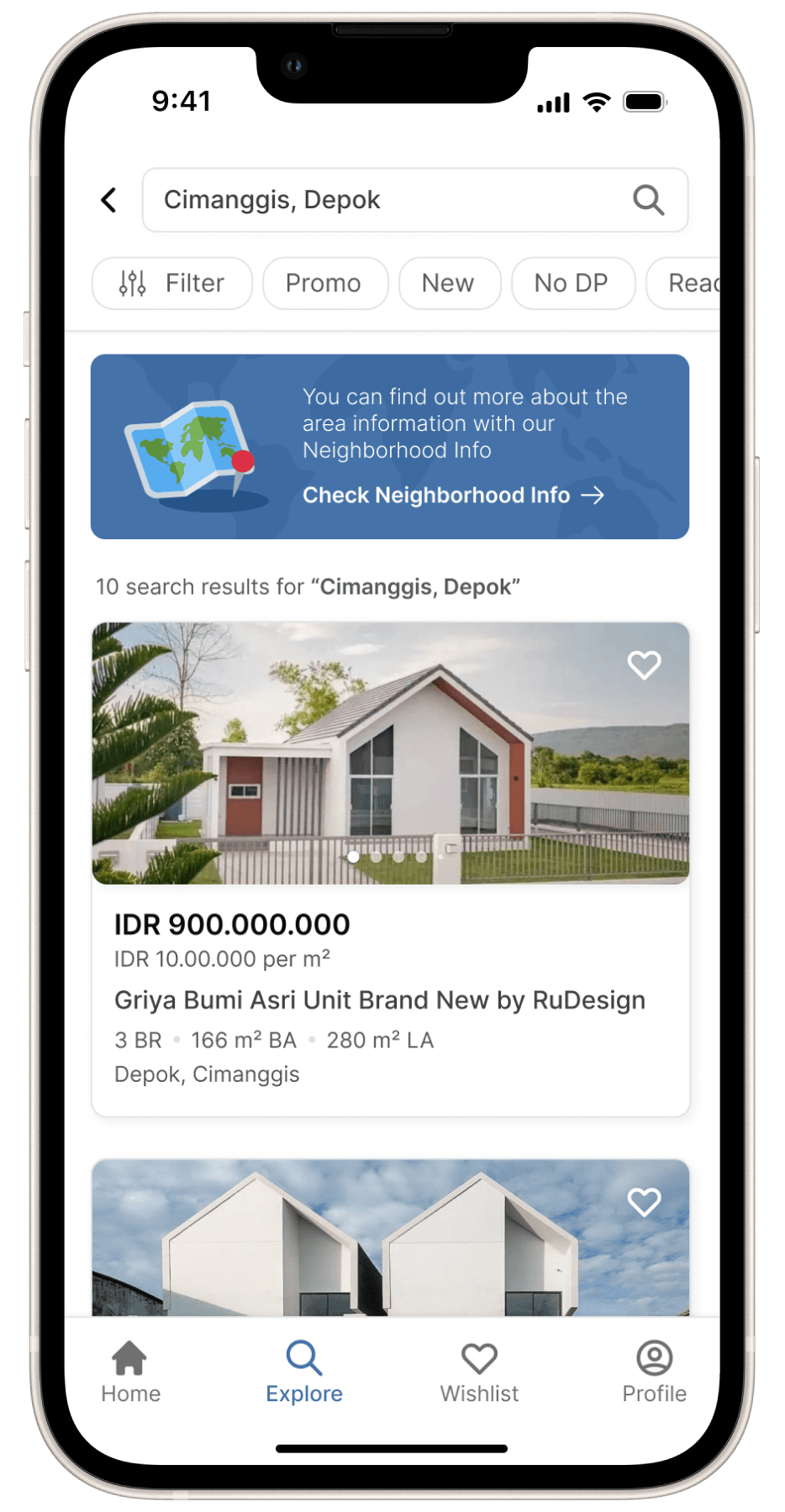The image displays a screenshot of a smartphone with a predominantly white background. 

In the top-left corner, the status bar indicates the time as 9:41, while the top-right corner shows full cell phone signal strength, full Wi-Fi connectivity, and a fully charged battery icon.

Beneath the status bar, on the left, there is a back arrow pointing left. Next to it is the search query "Semen niggas, Deepak." This name appears in the search bar, with the search icon situated on the far right of the bar.

Below the search bar are some partially visible categories: "Filter," "Promo," "New," "No DP," and a truncated word starting with "re."

Further down, a prominent blue box features white text and a map. The map uses blue and green colors, with a red pushpin indicating a specific location. The text within the blue box reads: "You can find out more about the area information with our neighborhood info check. Neighborhood info ➔."

Below the blue box, the text announces, "10 search results for 'Semen niggas, Deepak'."

Following this, there are images and details of houses. The first house is accompanied by text that reads: "IDR 900,000,000." Additional images and descriptions of houses appear underneath.

At the very bottom of the screen, a navigation bar displays icons for "Home," "Explore," "Wish List," and "Profile."